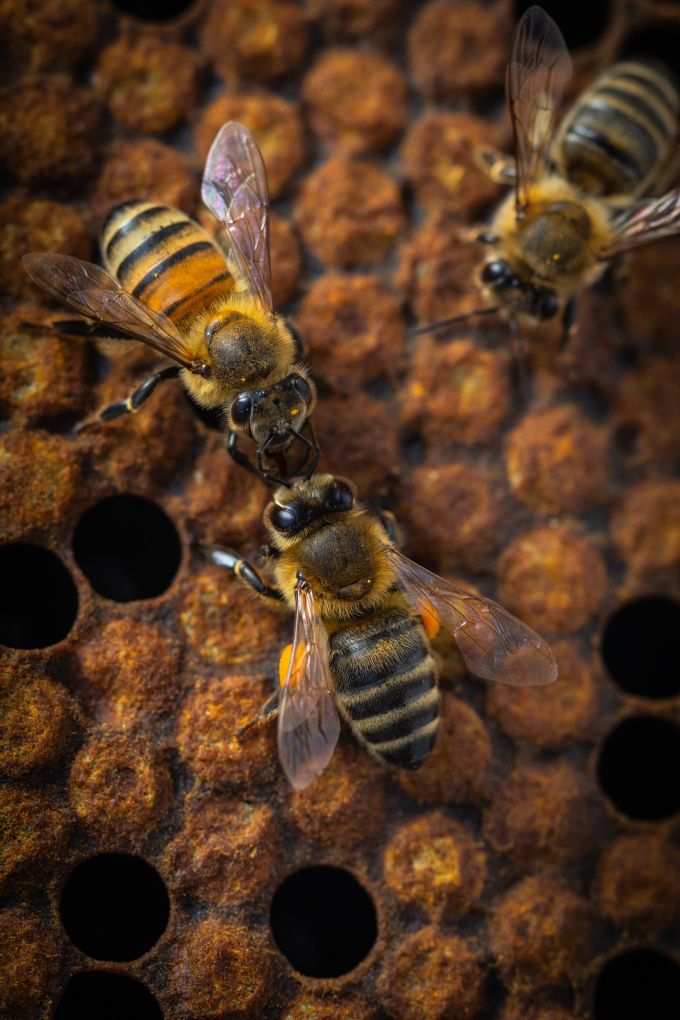The photograph is an extraordinarily high-resolution close-up of honey bees on a honeycomb. The honeycomb, colored in shades of yellow and orange with black accents in between the cells, is almost entirely capped, except for a few open cells. In the center of the image, two honey bees face each other, seemingly antenna to antenna. One of these bees, prominently in the center, has orange pollen stuck to the upper parts of its legs. The detailed resolution reveals the transparent texture of their wings, including the intricate veining, as well as the stripes on their fuzzy yellow and brown bodies. The lower right bee appears more yellow, while the upper left bee exhibits more black in its stripes. In the upper right corner, another bee, slightly out of focus, faces in their direction, adding depth to the composition. Their thin black legs with some yellow, resembling knees or joints, can be seen standing on the honeycomb. The image brilliantly captures the minute details, such as the variety in their stripe thickness and the clarity of their wings, making it an exquisite depiction of the bees in their natural environment.